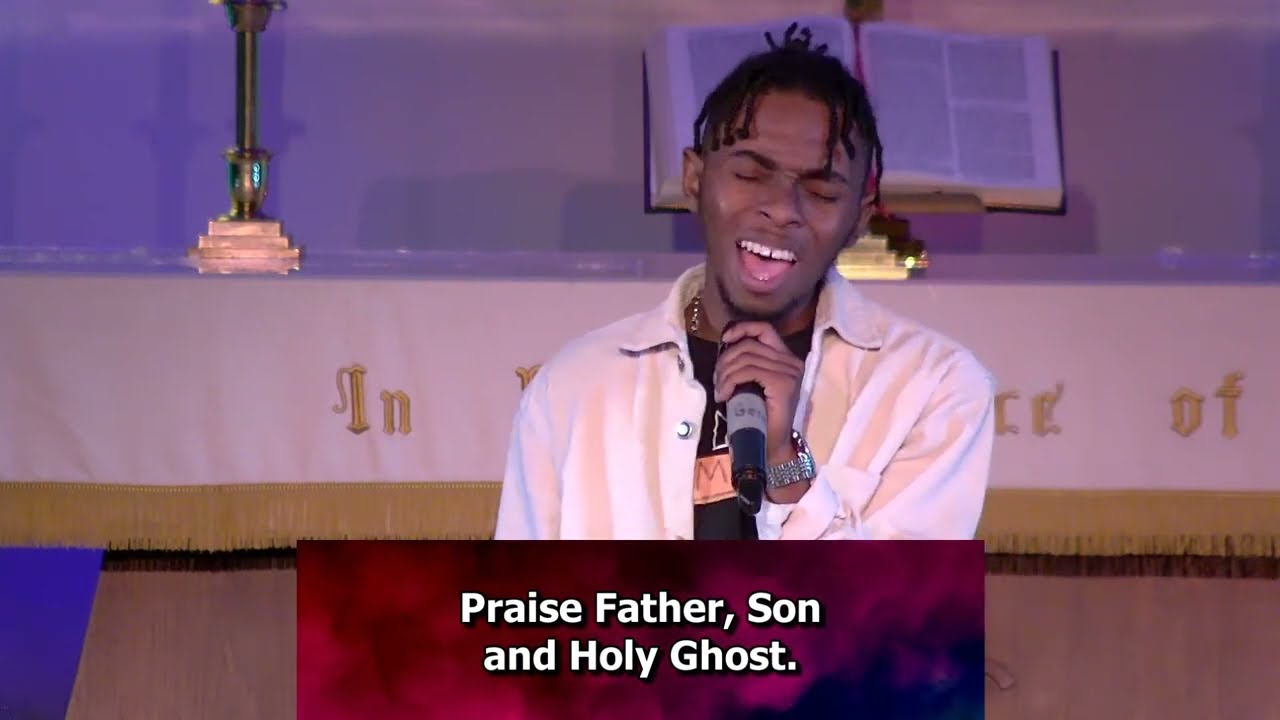In a church setting, a young African American man with short curly hair, accented by braids or cornrows at his forehead, stands passionately singing with his eyes closed and mouth wide open. Clad in a white shirt over a black t-shirt, a silver watch adorns his left wrist, and a chain hangs around his neck. He holds a microphone in his left hand. Behind him is a table draped with a tasseled cloth, embroidered with the partially visible words "IN…" and "…OF". An open book, likely a Bible, rests on a stand atop the table. To his front, a prominent red and purple banner displays the text "Praise Father, Son, and Holy Ghost", set against what appears to be hues of pink and blue clouds. Dim candlelight flickers beside the book, casting a serene glow in the background dominated by blues and grays.